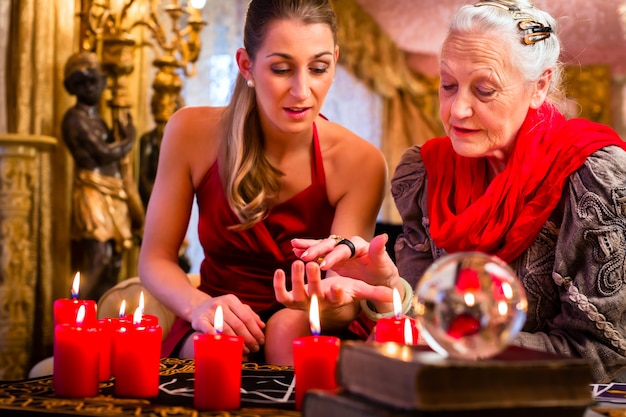In a luxurious setting adorned with opulent golden drapery, bronze statues, and elegant wall sconces, an evocative scene unfolds in an old-timey mansion. At the center of the image, two women are deeply engrossed in a moment of palm reading. The younger woman, in her thirties, sits on the left wearing a stunning red halter top dress, her light brown hair elegantly cascading over her shoulder. Her look is completed with delicate makeup and minimal jewelry, exuding a festive yet sophisticated charm, enhanced by the soft glow of the numerous red candles—eight or nine in total—illuminating the scene. 

Opposite her is an elderly lady in her seventies, with striking white hair adorned with tortoise shell barrettes, who has donned a beige-tan dress or jacket, complemented by a bright red scarf draped around her neck. With a serene expression, she carefully traces the lines on the younger woman’s palm, a crystal ball sitting on the table in front of her, hinting at her role for the evening. The background, slightly blurred, adds to the grandeur with intricate golden curtains framing a large window with lace details, contributing to the mystical and festive ambiance of the event. This captivating tableau suggests a sophisticated party where guests are treated to the enchanting art of palmistry.